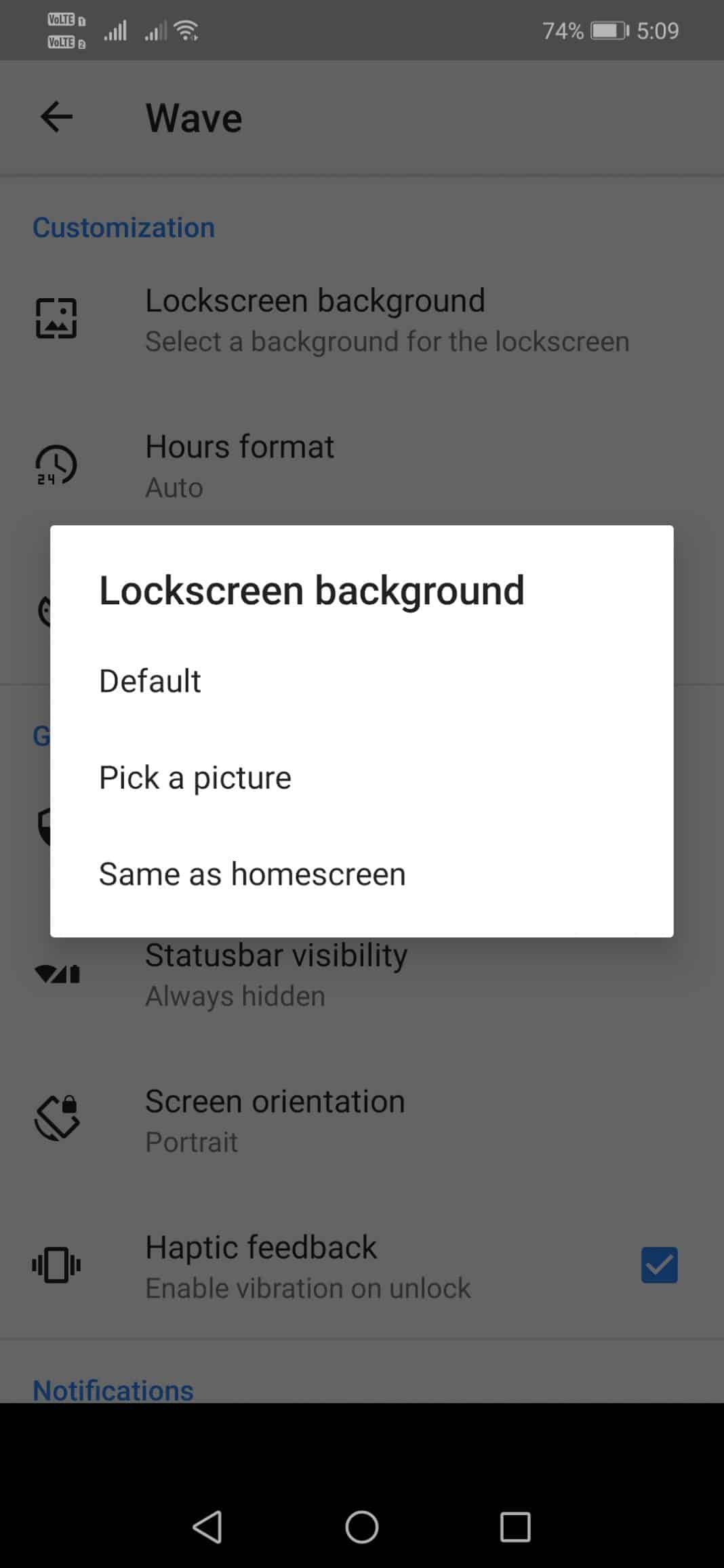A mobile device screen displaying various customization options is shown. The device has full WiFi connectivity and a 74% battery level with 510mAh remaining. Prominent on the screen is the WiIM application, offering customization features for the lock screen background. Users have the option to select a background image for the lock screen through an interface that includes options like "transform to auto" and "status bar visibility." The screen also allows toggling features such as portrait mode, active feedback, and optional feedback.

Blue squares with white numbers and notifications are displayed, alongside a black bar at the bottom indicating navigation icons: a sideways triangle, circle, and square. A window on the screen prompts the user to pick a picture for the lock screen background, with options to use the same image as the home screen background. The visible background is highly praised as a very great image. Further options include adjusting the format and visibility of the status bar.